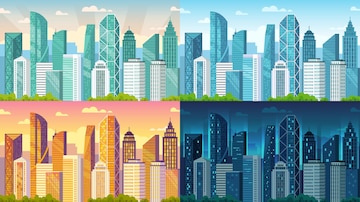The image is a vibrant, 3D-style cartoon graphic of a city, divided into four distinct sections, each representing different times of the day and color schemes. In the upper left section, you see a cityscape with mint green buildings against a clear sky with a few clouds and the tops of trees visible. This section has a touch of orange and a pinkish hue, indicating dawn. The upper right section depicts the same city but in a light blue color palette, with a sky that retains a white and blue tone with some clouds, suggesting daylight. The bottom left section illustrates the city during sunset, where the buildings are painted in orange, yellow, and purple shades, and the sky is a mix of purple, red, and yellow hues, reflecting a beautiful evening glow. Finally, the bottom right section shows the city at night, with deep, dark blue colors enveloping the buildings under a night sky. All sections feature a consistent city structure of tall high-rise buildings in the background and shorter structures with white trims in the foreground, emphasizing continuity across the collage.